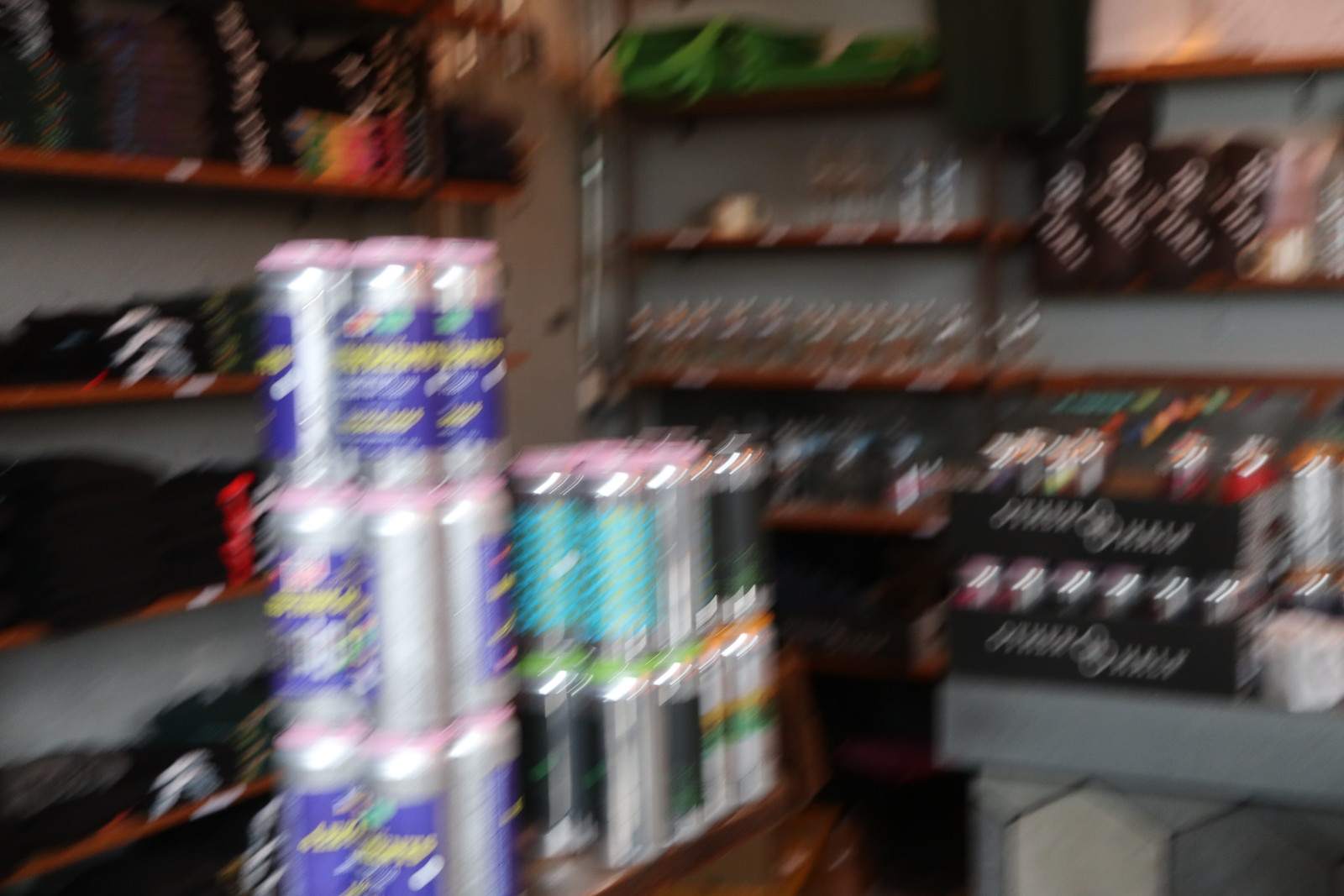The blurry photograph captures an indoor shop display, featuring industrial-looking shelves with silver racks and red or orange shelves. The scene is dominated by stacks of aluminum cans, which are largely indistinguishable due to the image's motion blur. These cans are adorned with a variety of colored stickers and labels—some are purple, aqua, gray, and blue, with hints of text that remain unreadable. The central display prominently features several organized stacks of cans arranged in three lines. Additional shelving to the left appears to hold folded black t-shirts and green tote bags. The overall disarrayed appearance of the photo creates an impression of a busy storefront, possibly a brewery, with its multitude of indistinct cans and colorful labels.